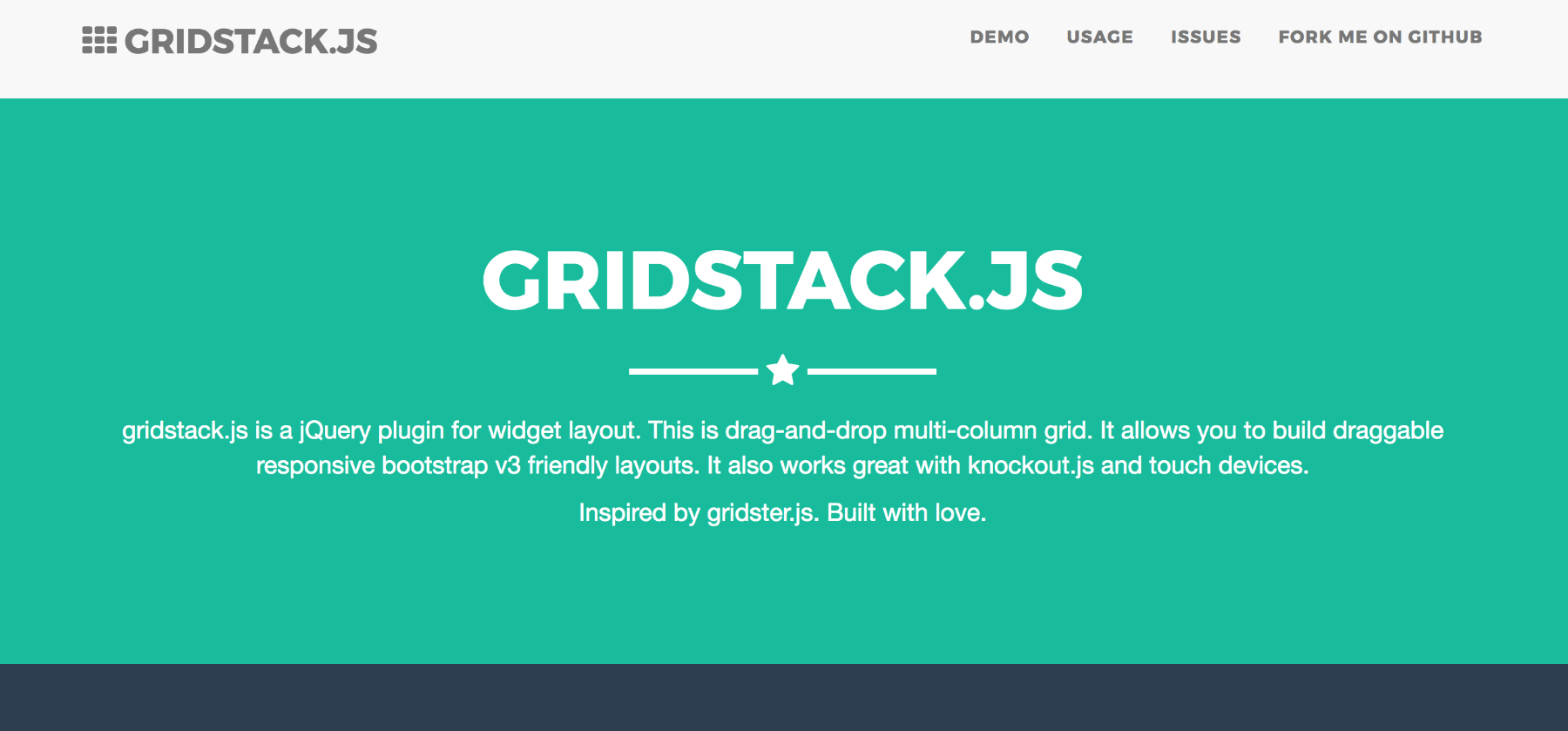A screenshot of a web interface features a green rectangular section with a gray header displaying the text "gridstat.js". To the left of the interface are three rows, each containing three square elements. The header also includes links for "Demo", "Usage", "Issues", and "Fork me on GitHub". Below the header, there is a line with a star icon in the middle, accompanied by the text "gridstat.js is a jQuery plugin for widget layout." The description elaborates that this tool supports drag-and-drop functionality within a multi-column grid, facilitating the creation of draggable, responsive layouts compatible with Bootstrap v3. Additionally, it integrates seamlessly with Knockout.js and is optimized for touch devices. Inspired by Gridster.js, this plugin is built with meticulous attention to detail.